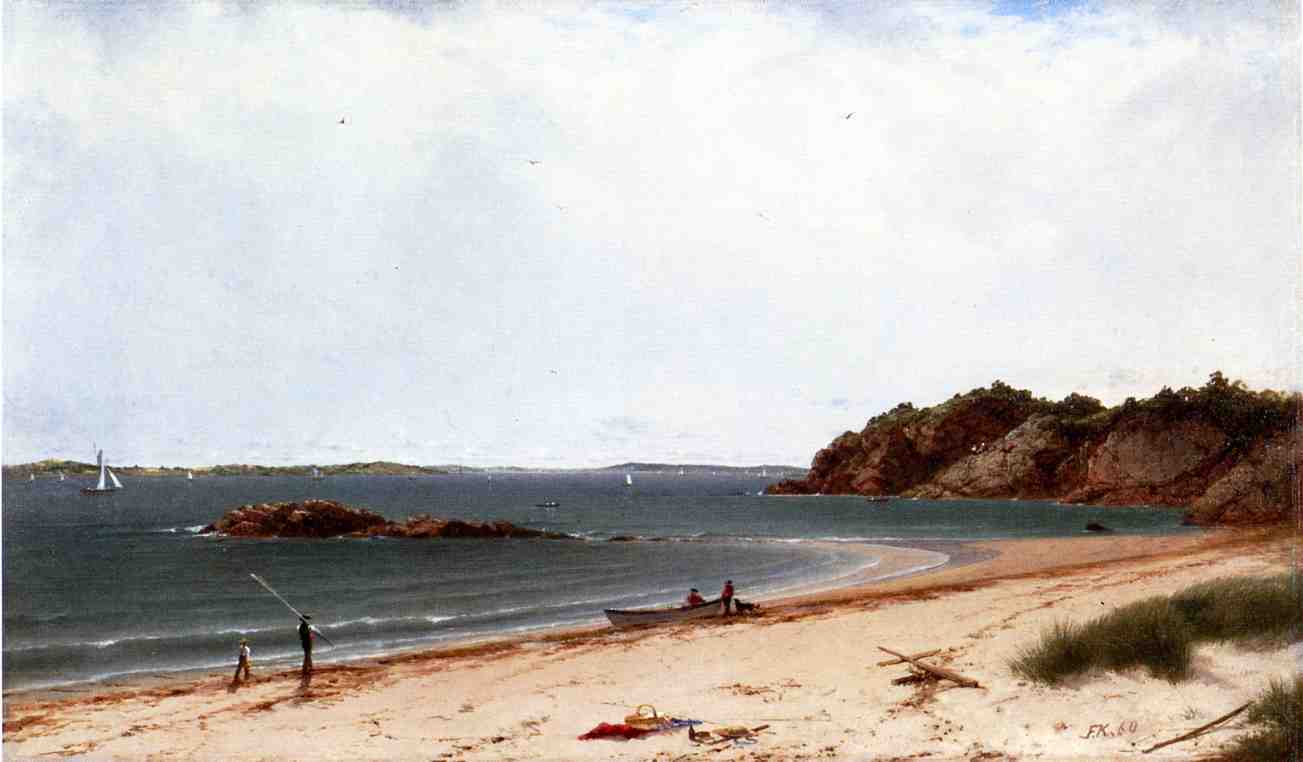This detailed oil painting, which could easily be mistaken for a photograph, captures a serene seaside landscape dominated by a light-blue, cloud-filled sky. At the forefront of the image, a light tan beach, realistically depicted with well-colored sand, stretches horizontally across half the painting, blending seamlessly into the dark teal waters. The beach is punctuated by tufts of gray beach grass and patches of driftwood.

In the center of the sandy shore, a distinctive red picnic blanket with a basket adds a touch of warmth to the otherwise muted palette. Nearby, a fisherman, equipped with a large pole, is seen walking alongside a child, presumably heading out for a day of fishing. Close to them, a small boat with two individuals is readying for its own journey into the water.

The rocky terrain features prominently on the right, with craggy outcroppings jutting into the sea, complemented by a small rocky island further out. Sailboats, their white sails visible in the distance, dot the water, adding a sense of activity and depth to the scene.

The sky, taking up a significant portion of the composition, is mostly overcast with fluffy white clouds, casting a soft, diffused light over the entire scene. This subdued lighting enhances the tranquility of the landscape, making the entire painting feel calm and picturesque.